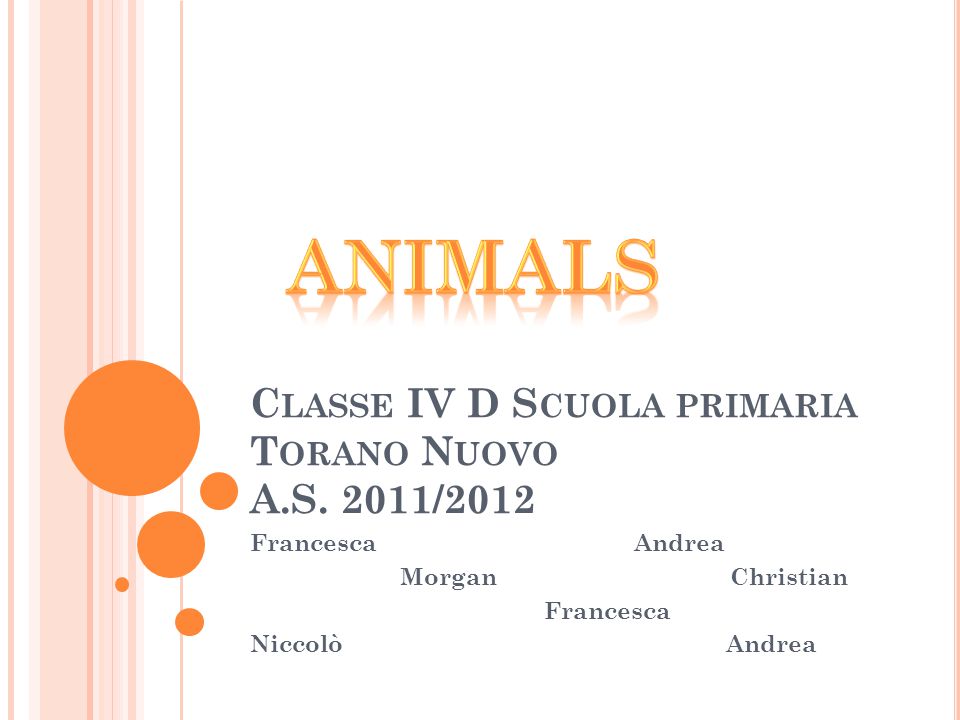The image is an advertisement or title page with a sleek, minimalistic design. It has a white background with intricate, vertically oriented colored lines along the left and right sides. The left side features an alternating pattern of thin pink and orange stripes, creating a gradient effect. In the top center of the design, the title "Animals" is prominently displayed in orange and yellow font, complete with a reflective effect that makes it appear as though it is positioned atop a shiny platform. Below this title are several brown and orange circles of varying sizes, reminiscent of planets arranged in a solar system. To the right of these circles, the text "Class IV-D, Scuola Primaria, Toronto, Nuovo, A.S. 2011-2012" is written in a bluish hue. Scattered below this text are the names of individuals involved: Francesca, Nicolo, Morgan, Francesca, Andrea, Christian, and Andrea. This layout evokes the look of a polished digital information screen or an opening slide of a professional presentation.